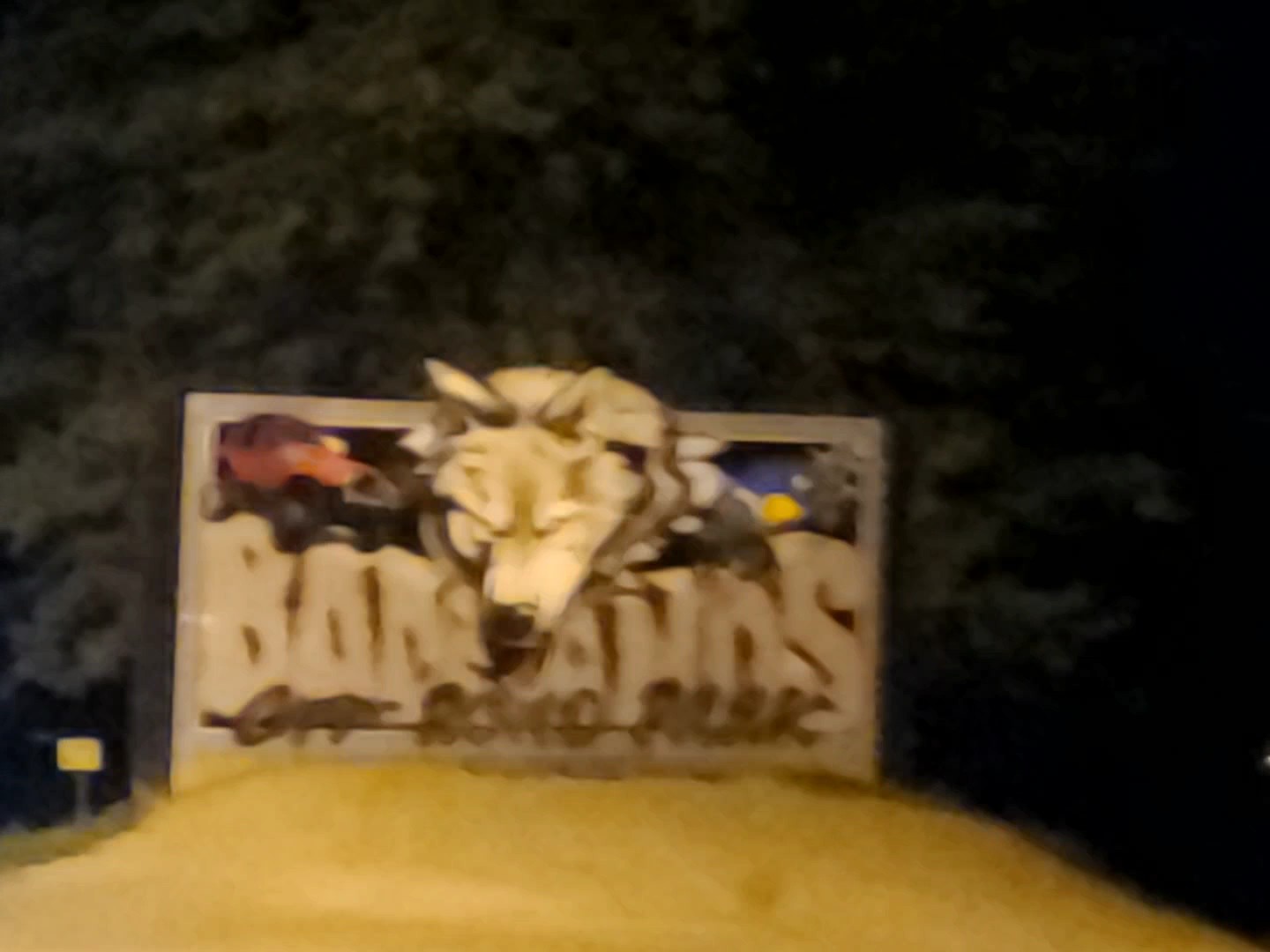This image, which appears blurry and low-resolution, depicts a nighttime outdoor scene featuring a rectangular roadside sign, possibly wooden, with a light tan border. The sign, resembling a billboard or vertical sign, is situated on a slight incline of sand or dirt and is partially obscured by the trunk and leaves of a nearby tree. The background is filled with dark green leaves under a dark sky.

At the center of the sign is a prominent, cartoonish wolf's head that aggressively peers over the top, its snout hanging over the word "Badlands," partially obscuring the letter "L." The text "Badlands" is styled to look like stone, and below it, there's partially obscured script and the word "Park," suggesting it is an advertisement for a park named "Badlands."

In the upper left corner of the image, a red Jeep with large black tires is visible in profile, overlapping the sign, adding a dynamic element to the scene. The sign and the mound of sand or dirt below it form the focal point of the photograph, capturing a rough, outdoorsy aesthetic.